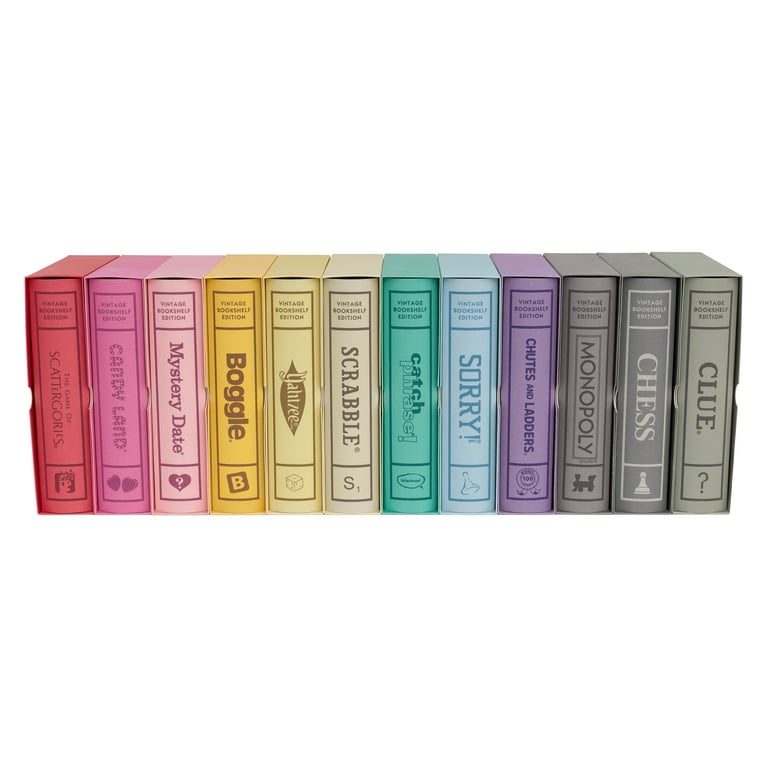This image showcases a collection of classic board games neatly arranged on a shelf, each enclosed in monochromatic, color-coded boxes that resemble book covers. From left to right, the games include Scattergories in a vibrant red box with darker red text, followed by a lavender-colored Candy Land box. Mystery Date comes next in a pinkish-peach hue, succeeded by Boggle in yellow and Yahtzee in a lighter yellow. Scrabble is presented in a greenish-yellow box, while Catchphrase appears in aqua green. Sorry is enclosed in a blue box, followed by Chutes and Ladders in purple, Monopoly in black, Chess in gray, and finally Clue in a lighter gray box. Each box features its respective game's logo in a matching, slightly darker shade on the front or side, enhancing the organized, bookshelf-like presentation against a white background.